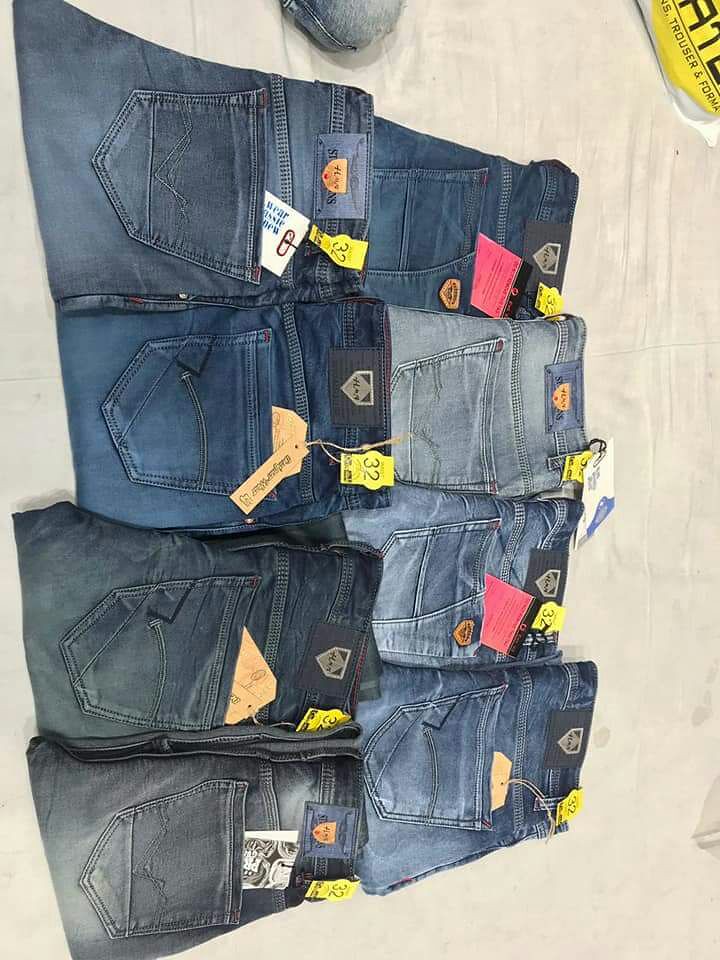This photograph, which needs to be rotated 90 degrees counter-clockwise for proper viewing, captures a neatly arranged display of eight pairs of folded jeans. The jeans, appearing slightly used, are arranged in two rows of four, with each pair folded to reveal only the waistband and back pockets. The variety includes dark blue, light blue, deep blue, grayish-blue, and black-blue jeans, potentially indicative of different washes or levels of wear.

Each pair of jeans prominently features tags: yellow cardboard tags reading '32', likely signifying the waist size, and additional tags in various colors—red, brown, and white—attached with traditional loops of string, with some tucked into the back pockets. These tags suggest the jeans might be in a commercial context, perhaps a store or a swap meet.

The background consists of a light ashen wood-effect flooring with visible grain running from left to right, reinforcing the retail environment feel. In the upper right corner, a hint of yellow and black fabric or material peeks into the frame, adding to the utilitarian and somewhat cluttered composition. This detailed and organized array of jeans, combined with the assorted tags and subtle background elements, suggests the image captures a commercial display, possibly in a clothing store or market setting.